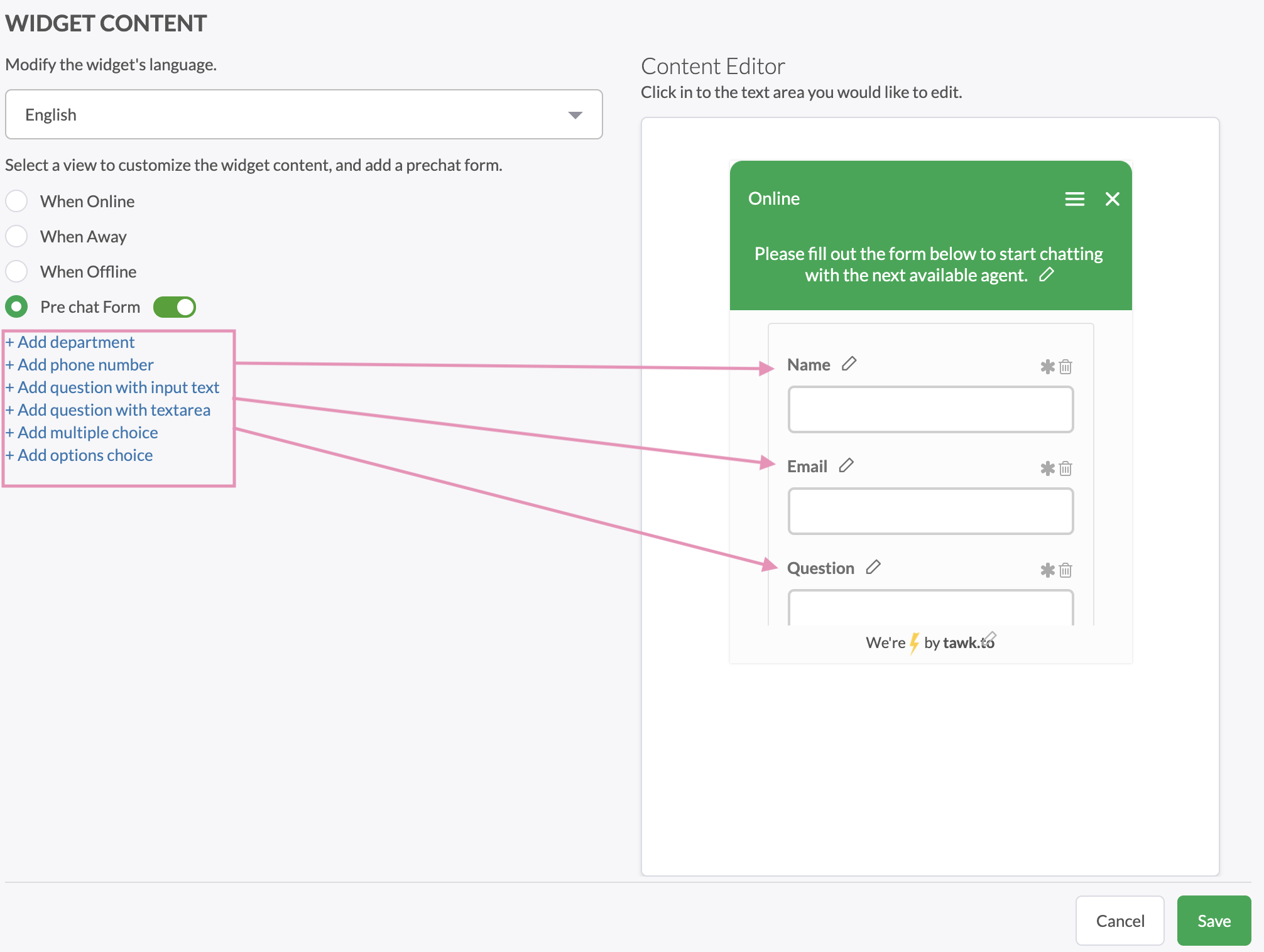The image depicts a detailed interface of a website called "Widget Content," focused on configuring a chat widget's language and behavior. 

On the left, the language is set to English, indicated by a drop-down menu. A message prompts users to customize the widget content and add a pre-chat form, with options such as "when online," "when away," "when offline," and "pre-chat form." The pre-chat form is highlighted in green.

Beneath this, a red box provides several options: "Add department," "Add phone number," "Add question with input text," "Add question with text area," "Add multiple choice," and "Add options choice." Three red arrows extend from this box to three white input fields labeled "name," "email," and "question," each accompanied by a crayon icon for editing.

Above these fields, a green box reads "Online" and contains instructions: "Fill out the form below to start chatting with the next available agent." Heading this section is the label "Content Editor," which guides users to click into the text area they wish to edit.

In the footer of the image, the branding "Whereby Hawk" is seen, featuring a yellow lightning bolt between "Where" and "by."